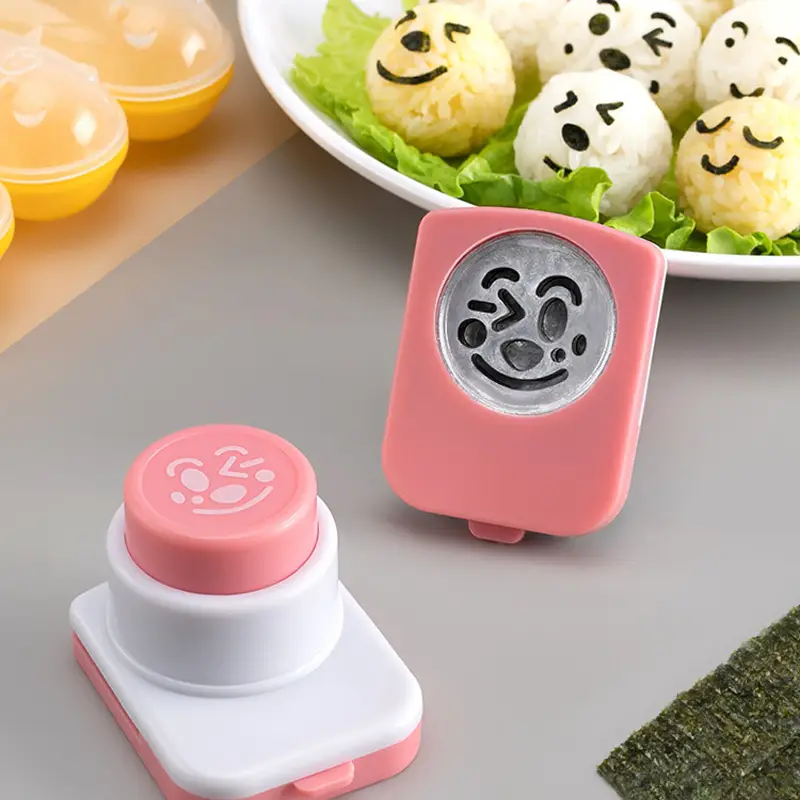The image features a vibrant and playful scene with various items centered around the theme of decorating food. In the top left corner, there's a yellow background showcasing two small, round yellow containers with clear plastic lids. To their right, positioned on a white plate, are five round rice balls — three white and two yellow — each adorned with cartoonish faces made of black shapes representing eyes, mouths, and eyebrows. One rice ball, positioned in the middle, interestingly features an arrow as part of its facial design. Below these rice balls, there's a pink-faced tool used for stamping faces onto the food, complete with a winking face and pimples on its cheeks. The lower left section of the image reveals a gray and peachy cupboard-like surface, with another accessory centered for stamping faces on food, illustrating the process of adding cheerful expressions to the rice balls. This close-up, color photograph captures the whimsical, happy vibes emitted by these colorfully decorated food items and their associated tools.